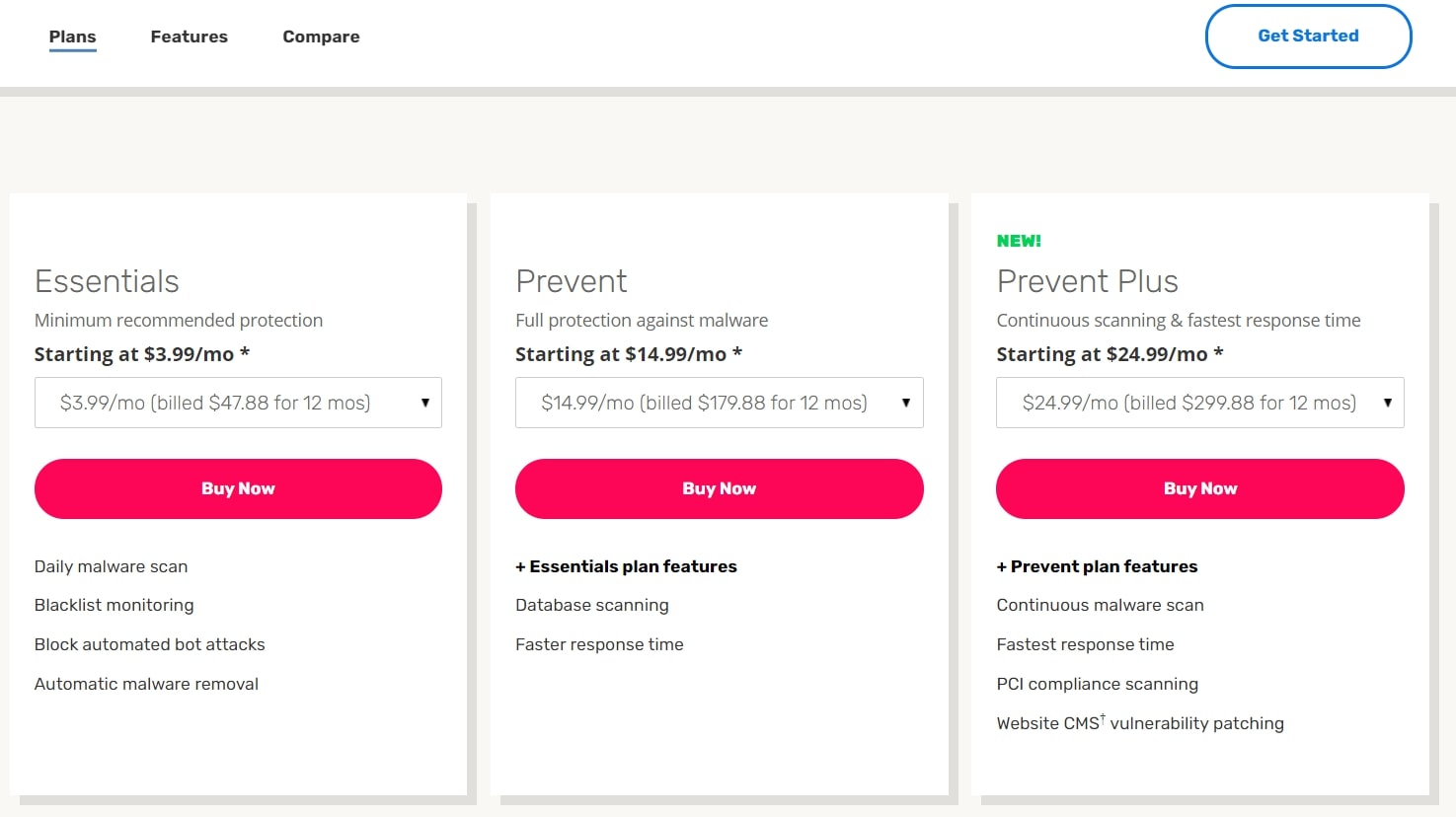This image shows a computer screen displaying a pricing and plans page for a software service. At the top, there is a navigation bar with several options: "Plans," "Features," "Compare," and a "Get Started" button highlighted in blue. The "Plans" section is currently selected, indicated by an underline beneath the word.

Toward the bottom of the screen, three colorful rectangles represent different subscription tiers, each featuring a "Buy Now" button in white text on a reddish-pink background. The plans are as follows:

1. **Essentials**:
   - Description: Minimum recommended protection
   - Price: $3.99 per month
   - Yearly Billing: $47.88 for 12 months
   - Features: 
     - Daily multi-malware scan
     - Blacklist monitoring
     - Blocking automated bot attacks
     - Automatic malware removal

2. **Prevent**:
   - Price: $14.99 per month
   - Yearly Billing: $179.88 for 12 months

3. **Prevent Plus** (marked "New" in green):
   - Price: $24.99 per month
   - Yearly Billing: $299.88 for 12 months